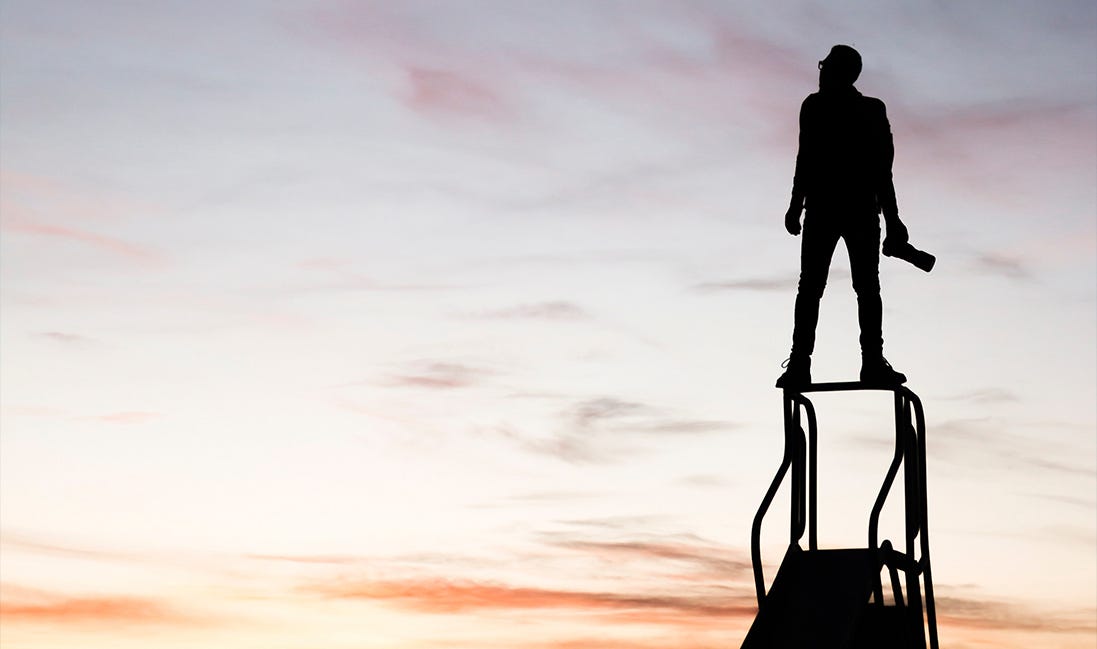The image captures the striking silhouette of a man standing confidently atop the precarious structure of a child's slide, framed against a hazy, multi-colored sky at either dawn or dusk. The sky is awash with a beautiful gradient of peach, pink, purple, and light blue hues, streaked with light clouds. The man, identifiable by his glasses and short hair, holds a large camera with a long lens, poised as if to capture the perfect shot. His wide stance and the precarious angle from which he stands, balanced on metal bars that resemble handles of the slide, add a sense of daring to the scene. Despite the precariousness, he appears focused and comfortable, with only his silhouette discernible in the softly lit background. The overall effect is one of serene yet precarious beauty, blending human focus and the ethereal quality of a twilight sky.